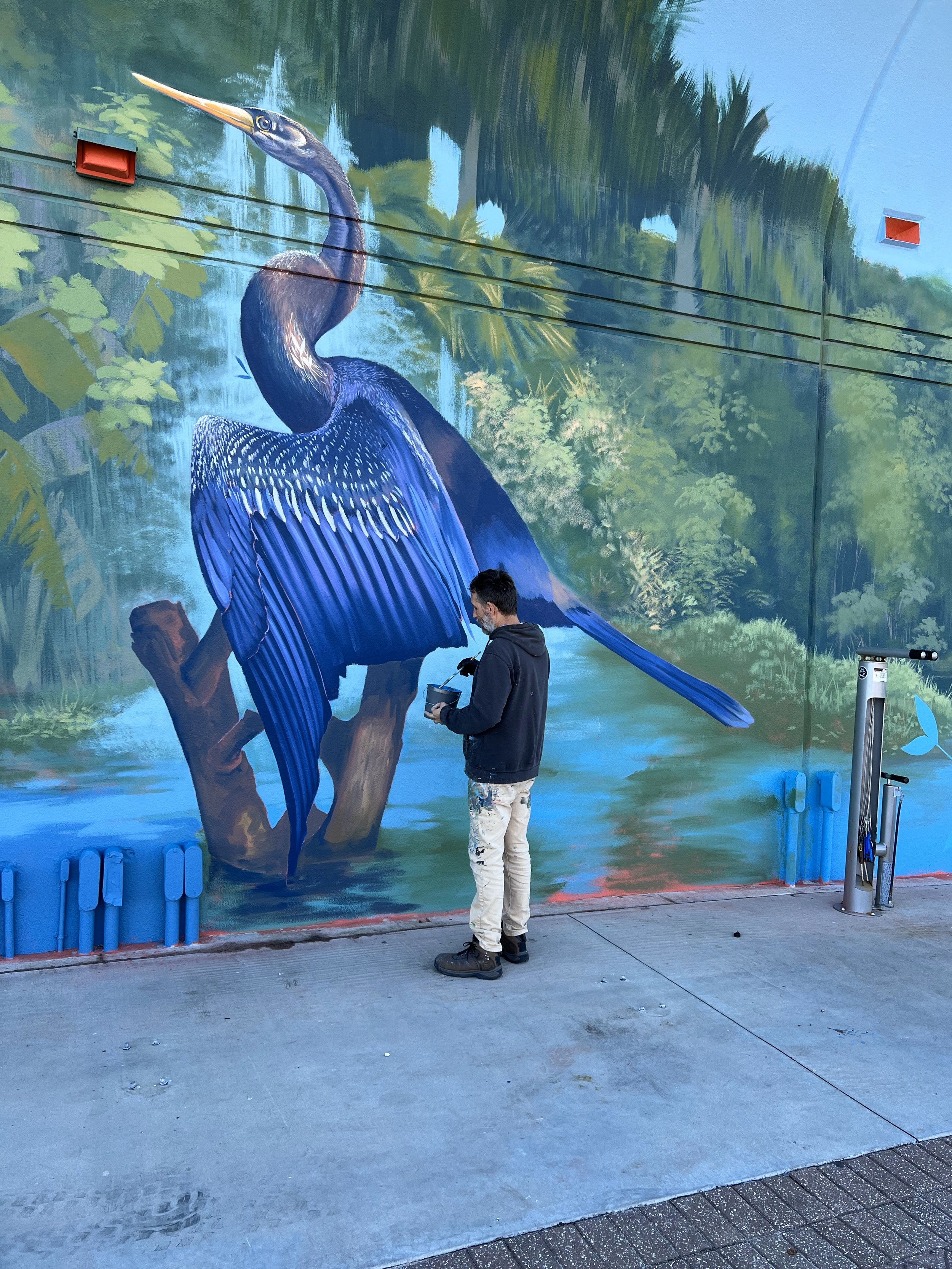This vertical color photograph captures a middle-aged man in the midst of painting an extensive mural on a large, slightly curved wall, possibly in a tunnel. The artist, clad in a navy or blue-gray hoodie with khaki beige, paint-splattered pants, and dark brown boots, is glimpsed from behind, angled to the left. His graying beard contrasts with his dark, almost black hair. The man is holding a silver paint can in his left hand, while his gloved right hand dips a paintbrush into it.

The mural itself is a vibrant depiction of a large blue heron, characterized by its long neck and sharp orange-yellow beak. The heron, which features striking blue plumage with touches of white, perches gracefully on a partially submerged branch in a richly detailed body of water. The background reveals a cascading waterfall amidst lush tropical foliage and vibrant, multicolored trees that extend to the right. The wall's curvature adds depth to the scene, and a gray sidewalk runs below the artwork, grounding the picturesque natural imagery in an urban setting.